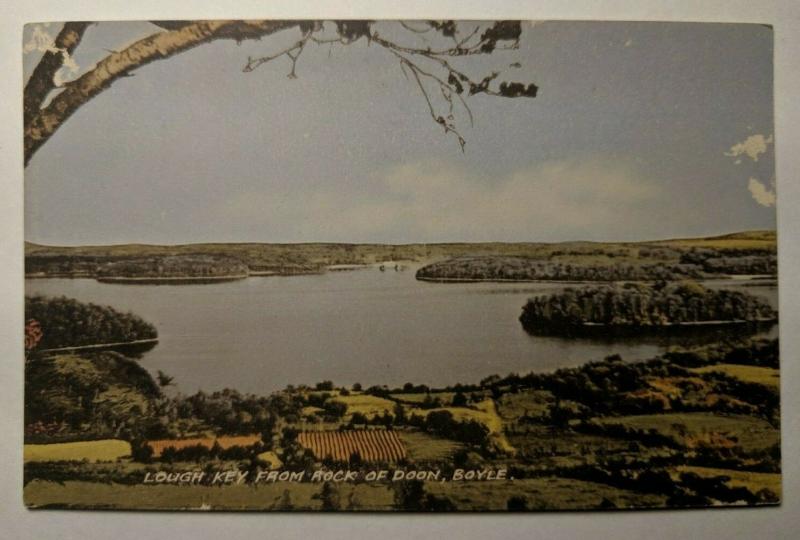The image is a photograph of an old, slightly faded and worn 4x6 photograph. The edges of the photograph are rounded and bent, with several scratches marring the surface. The photograph, taken outside during the daytime, features a scenic landscape by a lake, bathed in natural sunlight. In the bottom-left-hand corner, there are fields with rows of crops and scattered trees, their colors appearing dark green to nearly black due to the aged nature of the photo. The lake itself, a medium blue body of water, has a small, densely tree-covered island at its center. Across the lake, more vegetation and trees dominate the horizon, though there appears to be something indistinct in the distance, potentially boats. Wispy clouds float in a blue sky, and in the top-left-hand corner, a tree's branches and leaves jut into the frame. Superimposed in white text at the bottom of the image, it reads "Low Key from Rock of Dune, Boyle."